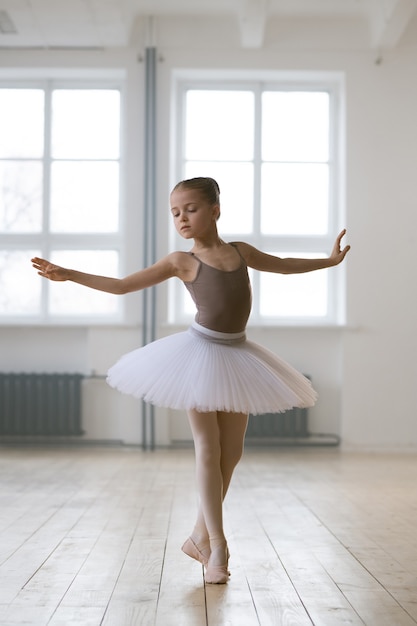The image showcases a beautifully illuminated, soft-focus photograph of a young ballerina, likely around six or seven years old, gracefully practicing a dance pose. She is elegantly attired in a sleeveless, brown or charcoal tank top and a white, frilly skirt known as a tutu that flares out above her knees. Her legs are covered by white tights, and she is wearing short ballet slippers. Her hair is pulled back, adding to her poised appearance. The ballerina has both arms outstretched, seemingly in the middle of a plié, and is gazing to the side, exuding an aura of elegance and focus. The setting is a serene, empty room with a plank wood floor, white walls, and two large windows that let in ample light. Beneath the windows, radiators run along the walls, contributing to the room's warm ambiance. The photograph captures this moment with a soft, blurred background that includes ceiling beams, all adding to the image's delicate and beautiful composition.